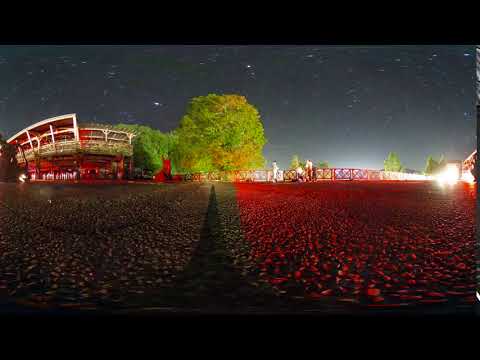The image is a vertical or rectangular shot taken at night, accentuated by horizontal black stripes across the top and bottom. The dark gray sky is punctuated with numerous tiny white stars, providing a serene backdrop. The field in the foreground has a reddish-gray cast, adding a mysterious ambiance. A dark gray walkway runs straight through the center, leading to a tall, lush green tree that stands prominently. The tree is very bushy with some brown leaves scattered atop and along the sides. 

To the left of this magnificent tree, there is a tall building with white rafters and railings on the top, its lower section predominantly red. Further to the left, and within the grounds, some trees grow around this structure. On the right side of the image, there's a low, possibly red and white fence line, behind which more green trees are visible. Flower gardens are also present, with beautiful red flowers covering one side of the ground, and light pinkish flowers on the other, all well-lit despite the nighttime setting. 

Overall, the image portrays a scenic environment blending natural and man-made elements, illuminated under a star-studded night sky.